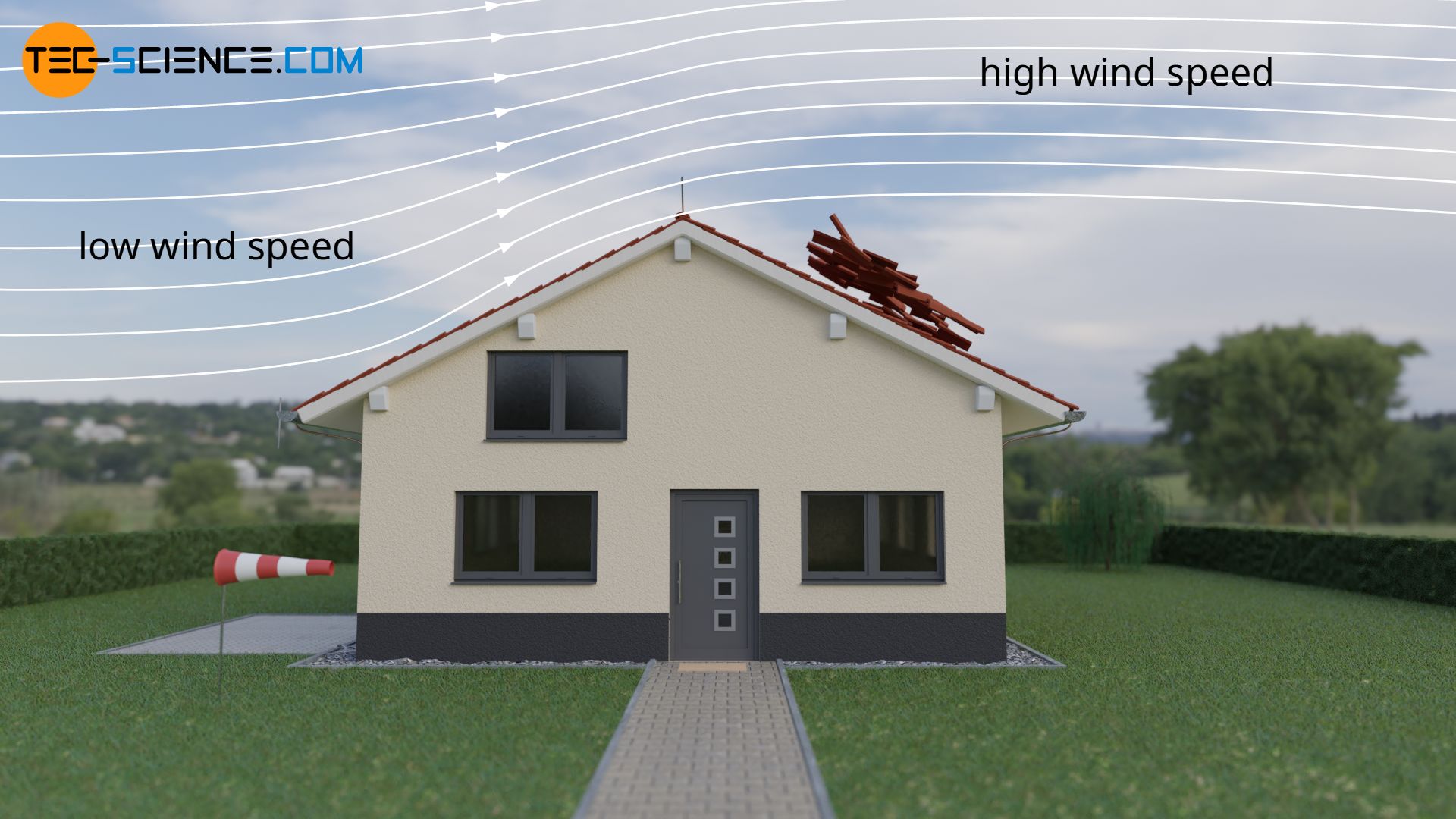This computer-generated drawing serves as a visual aid to demonstrate wind speeds around a house. Centered in the image is a two-story cream-colored stucco house with a slate blue door featuring four small square windows. The house is framed at the base with gray trim and has one window on either side of the door, plus another window on the second story to the left. A cobblestone walkway leads up the middle of a digitally green lawn to the front door. A row of hedges borders the yard on both the left and right sides, extending behind the house.

To the left of the house, a red and white striped windsock on a pole indicates wind blowing to the right. The house has a pitched red roof, and a bundle of wood or debris is visible on the right side of the roof. The illustration includes eight or nine white wavy lines over the roof to represent wind patterns. On the left side of the roof, the lines are labeled "low wind speed," while on the right side, where the lines rise, they are marked "high wind speed."

In the background, a hillside dotted with houses can be seen on the left, along with some trees and grass. To the right, there is open grassland and distant trees. The upper left corner of the image features the logo "TECsience.com" with the "TC" in a yellow circle and "science.com" in black text, illustrating the source of the educational content.